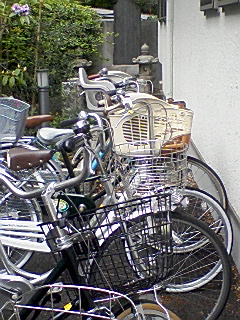The image is a horizontally-oriented, small, and somewhat poor-quality photograph depicting a row of bicycles parked against a white stucco wall. The bicycles, numbering three or four, are aligned in a row and all face towards the right side of the image. Each bicycle features a front basket, with some being made of plastic and others metal, showcasing a mix of vintage and modern styles. The seats appear to be leather, while the wheels are predominantly black, except for one which has a touch of white in the center. 

In the background, on the upper left side, there is a lush green tree or shrub, providing a contrast to the stark wall. Below the foliage, a small, hip-high lamp post or streetlight is visible. Additionally, there is a gray object, potentially a window, situated in the upper right corner of the image. A classic Zen lantern and a dark gray cement structure are faintly discernible towards the central background of the photo. The ground beneath the bicycles comprises a blend of concrete and dirt.